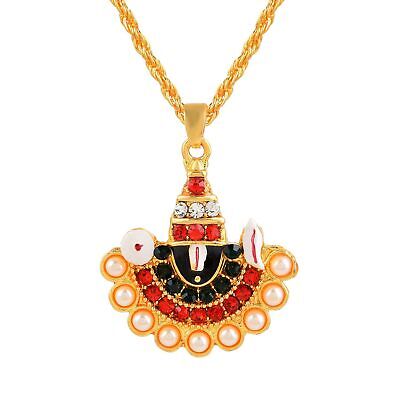This photograph depicts an exquisite necklace featuring a thick, gold rope chain that culminates in a V-shape. Attached to the chain is a luxuriant pendant that begins with a triangle formation of gemstones: one red stone at the peak, followed by a row of three white diamonds, succeeded by a row of three red rubies. Below this section, the pendant fans out into an upside-down semicircle adorned with a central black stone, flanked by eight smaller black stones that outline the arch. Encircling these are nine rubies, followed by nine delicate pearls, all set against a backdrop of gold that borders the entire pendant. Additionally, there appear to be subtle shell-like details within the design.